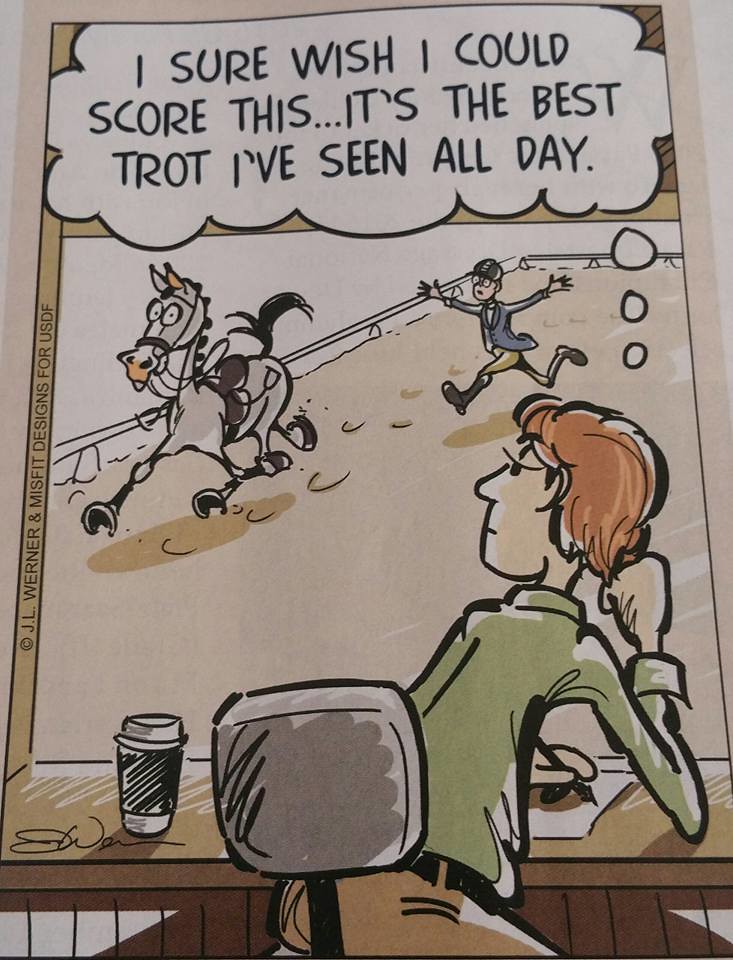In this horizontally oriented, rectangular comic strip cell, a woman is depicted sitting at a table, leaning onto the surface in a comfortable yet somewhat concerned pose. Dressed in tan pants and a long-sleeved green shirt, she sits on a gray-and-black office chair, with her right elbow propped on the table and her chin resting on her fist. A takeout coffee cup with a darker sleeve sits nearby. 

The scene she observes through a large window reveals a comedic moment: a bewildered gray horse with wide eyes is running left within a white-lined, tan-floored corral. The horse is saddled and harnessed, pursued by a frantic rider dressed in traditional British jockey attire—knee-high black boots, tan pants, a blue jacket, and a brimmed jockey hat—both arms outstretched trying to catch the runaway horse. 

The woman's thought bubble, positioned near the top of the image, reads in all caps, "I sure wish I could score this. It's the best trot I've seen all day." The left edge of the comic features the copyright notice "© J.L. Werner and Misfit Designs for USDF" in black letters, with additional white panels in the bottom-left corner.